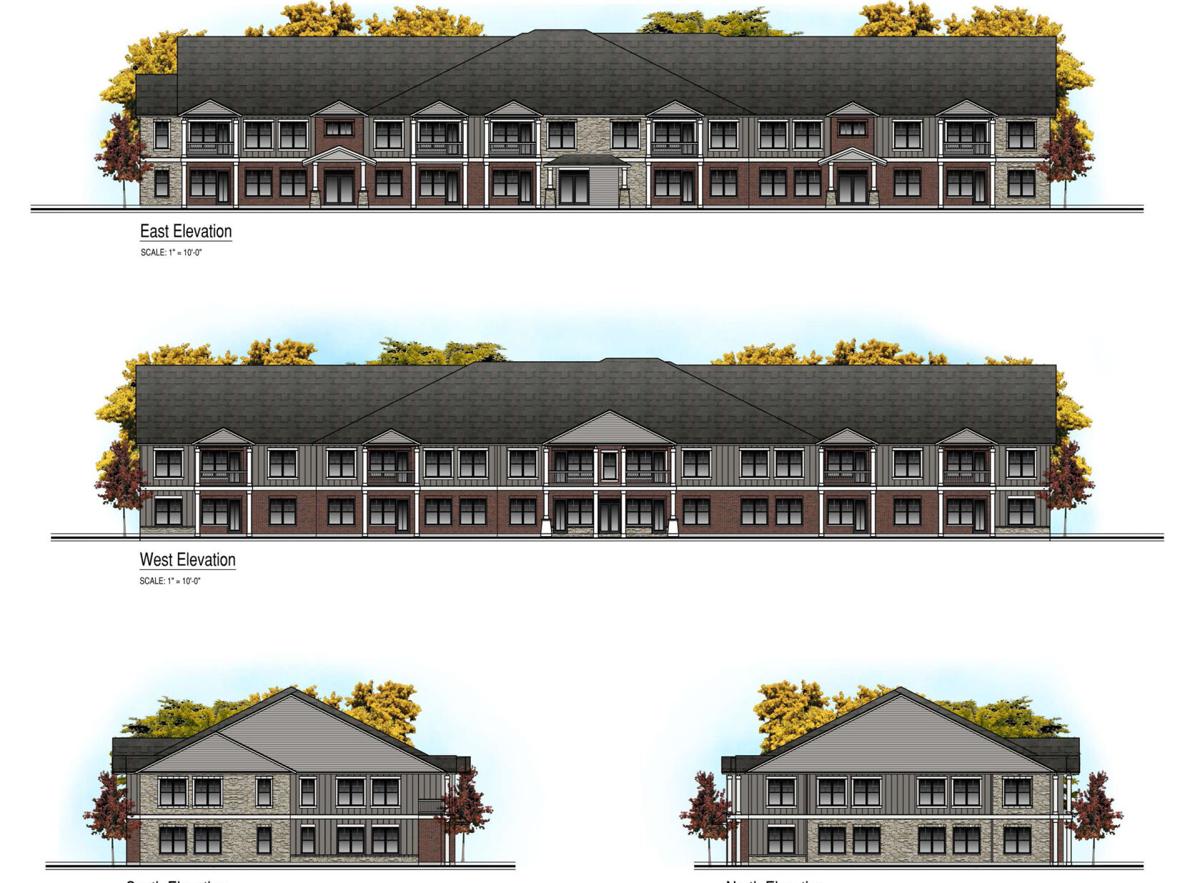The image features computer-generated architectural drawings of a two-story building with gabled roofs, set against a white background. The drawings are arranged in three rows, each depicting different elevations of the same structure.

In the top row, labeled "East Elevation" with a scale of one inch equals ten feet, the drawing showcases a wide, two-story building with gray gabled roofs, porches on the ground level, and balconies on the upper floor. Flanking the building are trees, visible on both the left and right sides, as well as above the roofline. The structure resembles a large residential house or a motel due to its expansive layout and detailed features.

The middle row presents the "West Elevation," also scaled at one inch equals ten feet, illustrating the same building. This elevation mirrors the details of the East Elevation, including the two-story height, gabled roofs, and the arrangement of porches and balconies. The façade appears to have a different color scheme, with brown on the bottom floor and gray transitioning to black at the roof.

In the bottom row, a pair of drawings likely depicts the side views of the building, emphasizing the gabled roofs and the two-story configuration with a porch on the ground floor and a balcony above. These side elevations lack textual labels but provide additional perspectives, completing the architectural documentation of the building.

All elevations include small glimpses of the skyline, enhancing the sense of scale and context within the architectural renderings.